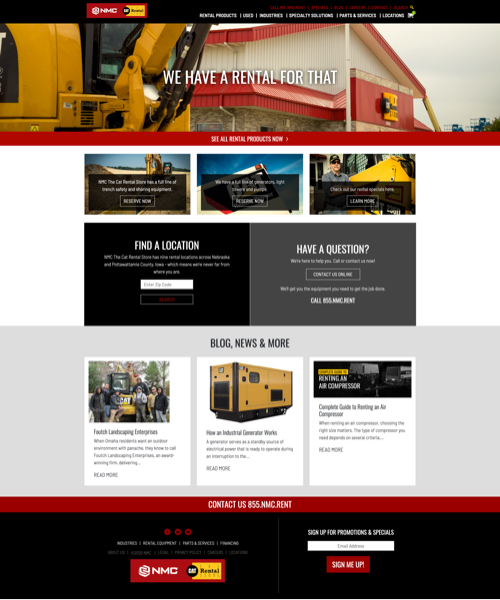The website for NMC, a heavy equipment rental company specializing in heavy construction machinery, features a prominent logo. The homepage boasts a banner at the top displaying the phrase "We Have a Rental For That," accompanied by an image of a bucket loader. The central and lower sections of the page offer various functionalities, including an option to find the nearest rental location by entering a zip code, and a support button labeled "Do You Have a Question?" for customer inquiries. Near the bottom, the site provides sections titled "Blog," "News," and "More," likely encompassing industry news, company updates, new equipment releases, and potential product recalls. Additionally, visitors can enter their email address to subscribe to the company's newsletter and receive updates.